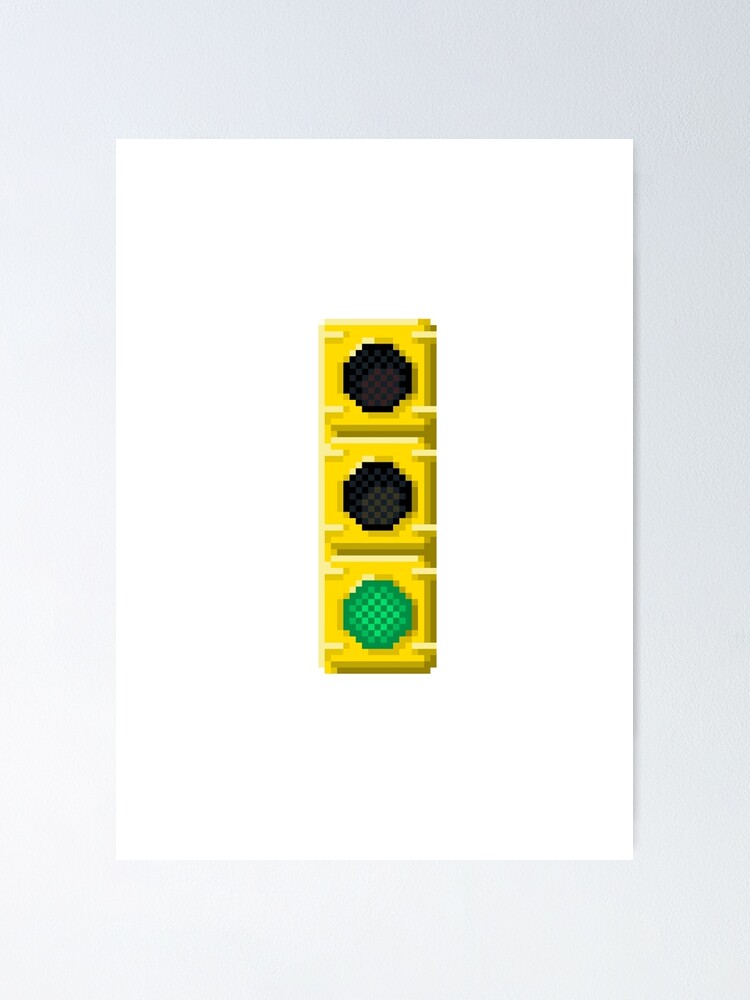The image is a computer-generated rendering of a rectangular stoplight with a cartoonish, pixelated appearance. The stoplight is depicted in a digital frame pattern, with the outer frame being a light gray tone and an inside matte of white. The stoplight itself is yellow and consists of three circular lights arranged vertically. The top and middle lights are black and not lit, while the bottom light is lit green, indicating "go." The pixelated details of the lights and the overall design give it a somewhat fuzzy, video game graphic look. The yellow stoplight is centered against a white rectangular background, which in turn is set against a larger, slightly gray background. No text or signature is present in the image, and the color palette includes shades of yellow, green, gray, black, and brown.